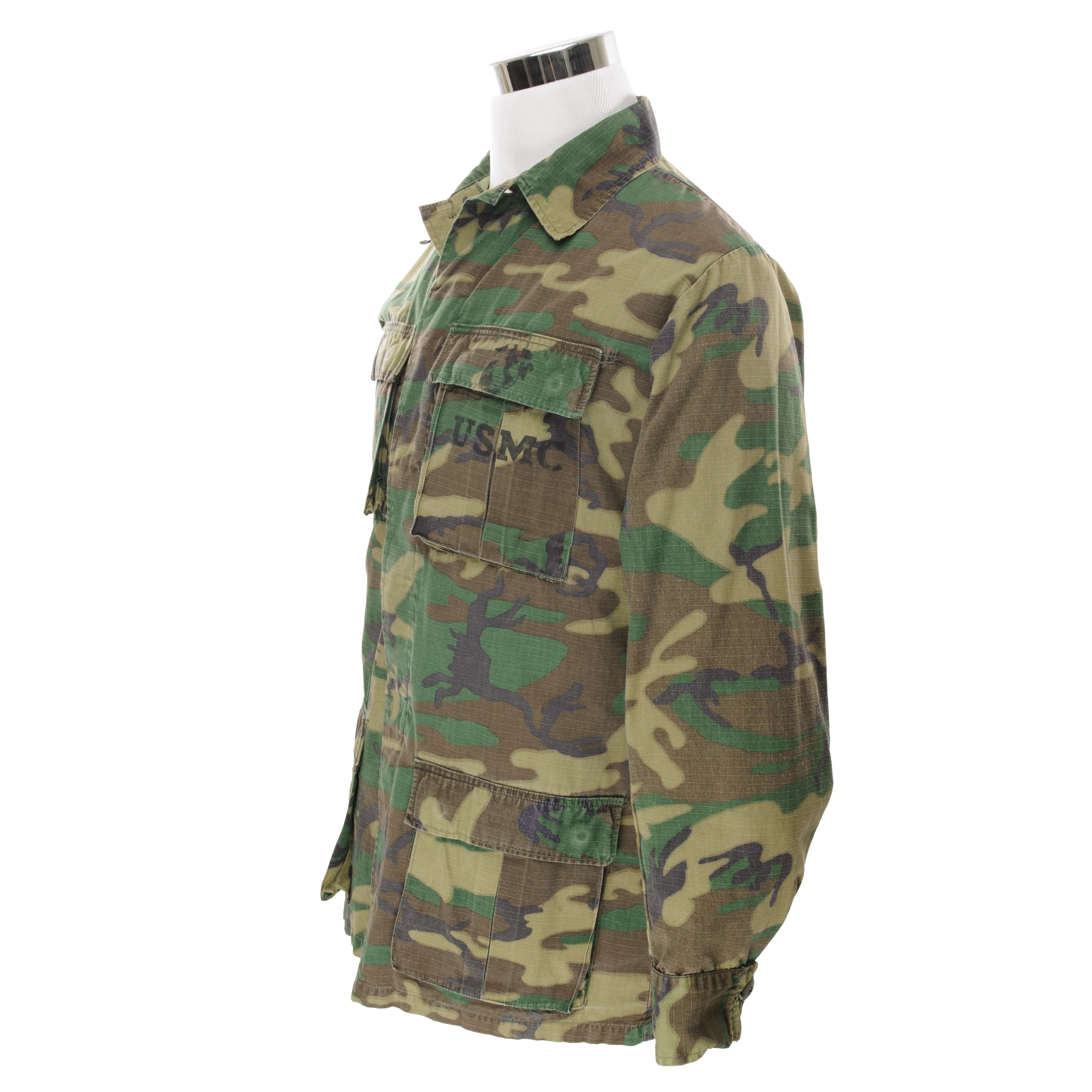The image displays a white mannequin torso with a silver cylinder through the middle, draped in a long-sleeved military camouflage jacket. The jacket has a classic green, black, brown, and tan camouflage print and features the letters "USMC" on the left breast pocket, indicating it is a United States Marine Corps uniform. There are four buttoned pockets on the front—two on the chest and two lower down. The collar is buttoned down, and the sleeves are cuffed with buttons at the ends. The mannequin is positioned facing slightly left from the viewer's perspective. The background is undefined and plain white, emphasizing the showcased jacket.